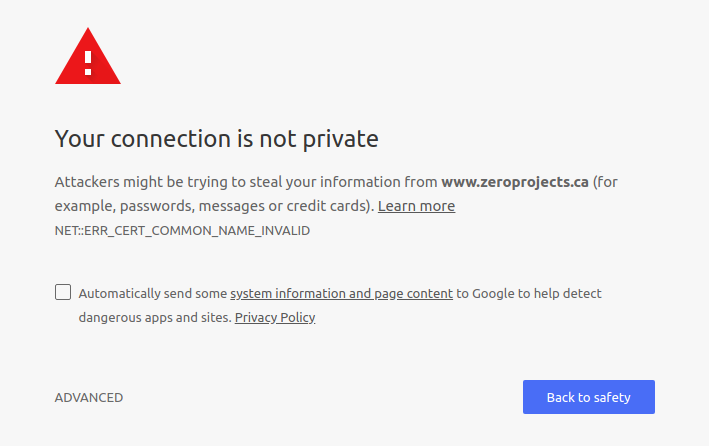In the image, there is a pop-up warning commonly encountered on the internet, alerting users about potential security risks on a website. At the top of the warning, there is a prominent red triangle with a white exclamation point inside, serving as a caution symbol. Just below the triangle, the warning message is displayed in large, bold font stating, "Your connection is not private."

In smaller text beneath the main warning, it explains, "Attackers might be trying to steal your information from zeroprojects.ca. For example, passwords, messages, or credit cards." There is a clickable link labeled "Learn more" that likely provides additional information about the warning.

Additionally, the warning includes a technical error message, "NET::ERR_CERT_COMMON_NAME_INVALID," indicating a specific issue with the website's security certificate.

At the bottom of the warning, smaller text mentions, "Automatically send some system information and page content to Google to help detect dangerous apps and sites." To the right of this, there is a blue clickable button labeled, "Back to Safety," allowing users an easy way to navigate away from the potentially harmful site.